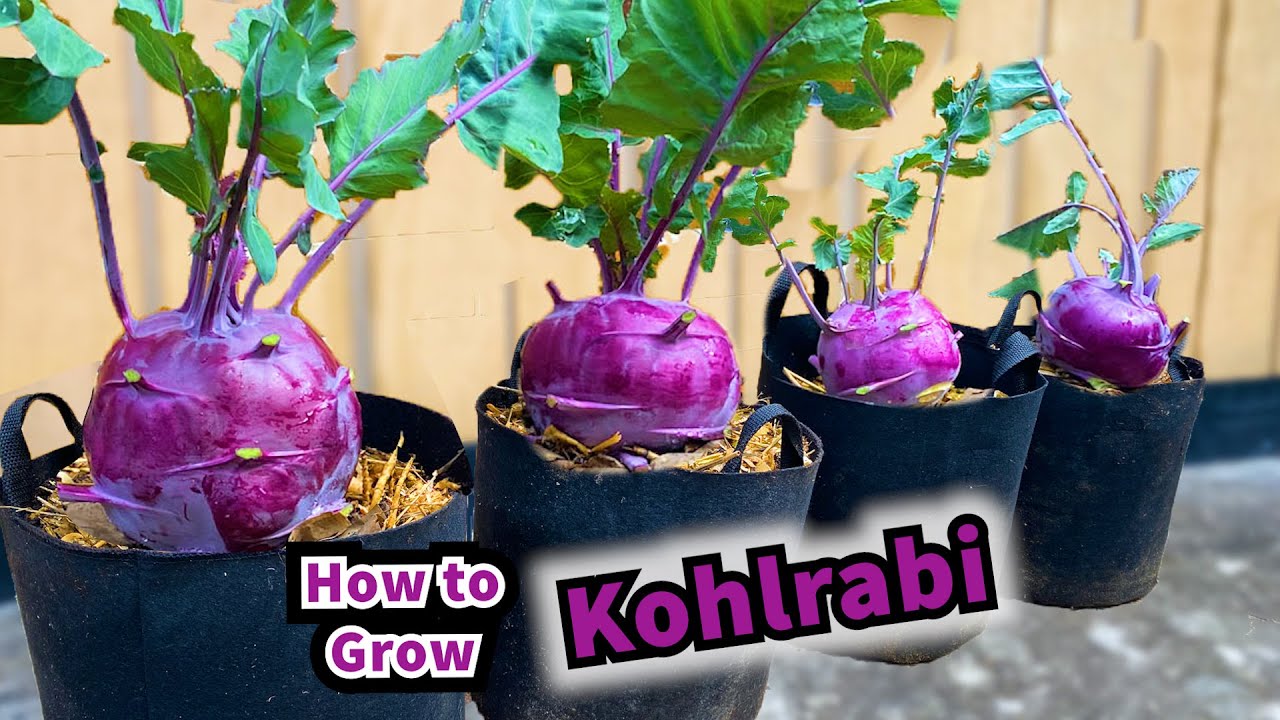This image appears to be a thumbnail for a YouTube video or cover image for a related article on how to grow kohlrabi. The centerpiece of the image features four large, purple kohlrabi plants with vibrant green leaves emerging from black containers. These containers are filled with what looks like light brown straw or hay, placed on a surface that appears to be a cement floor. The background shows a brownish hue, possibly indicating a fence or some other slightly out-of-focus structure. The text "How to Grow Kohlrabi" is prominently displayed on the image. "How to Grow" is written in purple letters with a white outline, and the word "Kohlrabi," also in purple, is embossed in black with a subtle white shine. This visual clearly intends to guide viewers or readers on the process of cultivating kohlrabi, emphasizing both the beauty and the method of growing this distinctive vegetable.